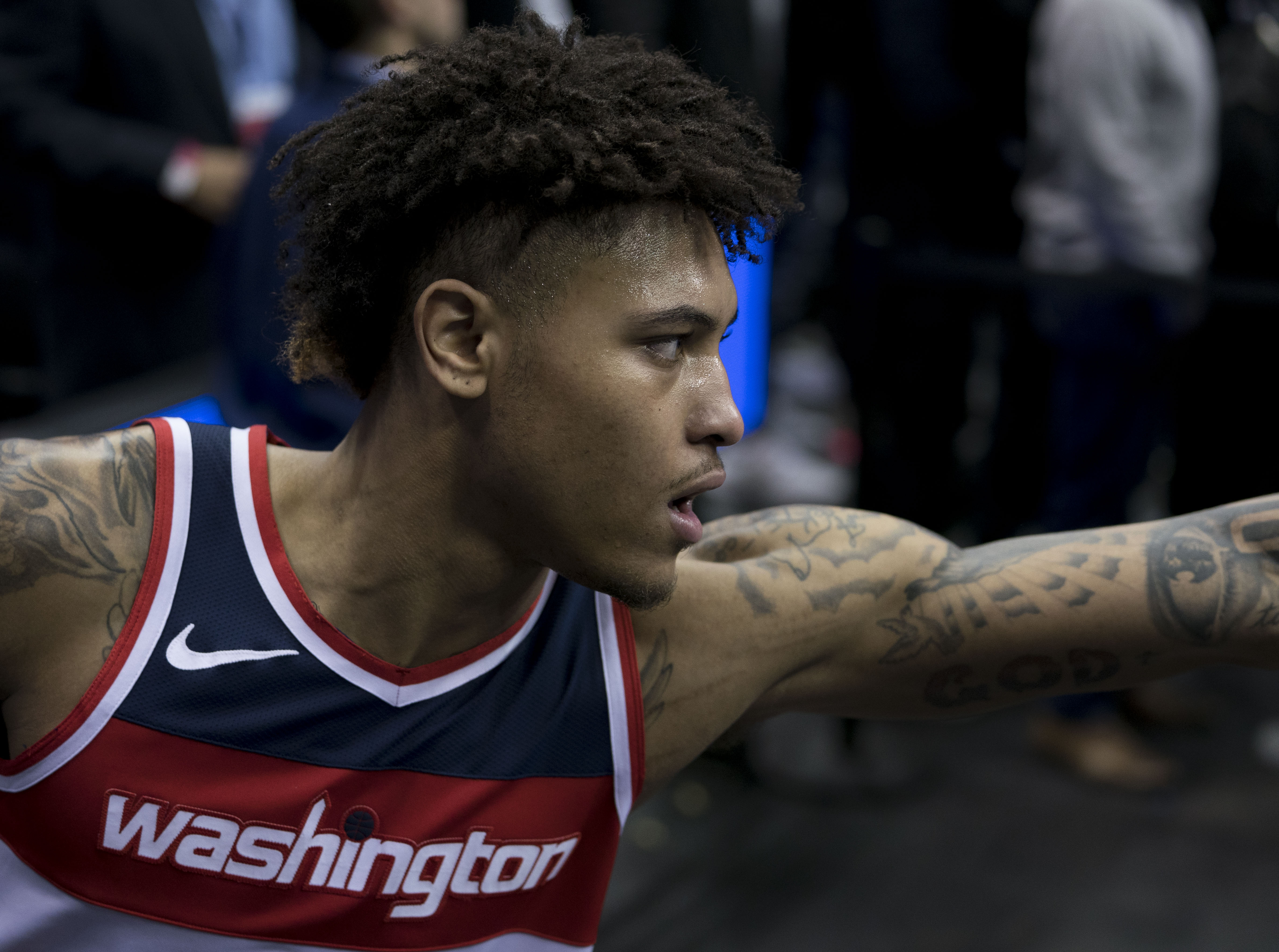The image captures Kelly O'Bray Jr., an athlete in the midst of a live basketball game. He is wearing a distinctive blue, red, and white jersey featuring a white Nike logo and the word "Washington" across the front in bold white letters. The jersey has red borders, complementing its tri-color scheme. Kelly's left arm is outstretched, displaying his well-defined muscles and numerous tattoos that extend from his shoulders down to his arms. His hair is a mix of short shaven sides and poofy, short dreadlocks on top. He sports a thin mustache and a bit of chin hair. Kelly is looking to his right, seemingly focused on the game. The background is blurry, with various onlookers likely watching the live action unfold.